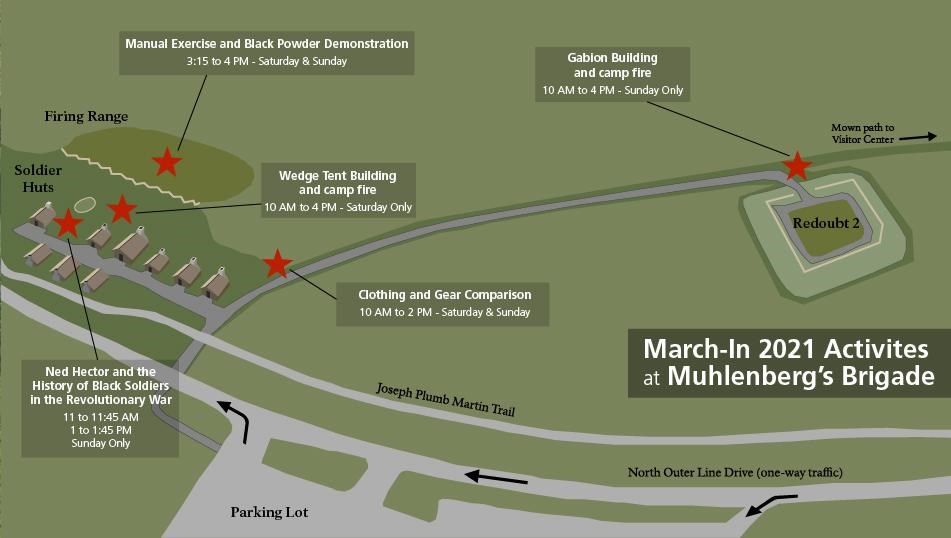This computer-generated illustration is a detailed, albeit not to scale, map of the Muhlenberg Brigade activity area. The diagram highlights the layout of the grounds, pinpointing key locations and events. Notably, it marks the parking lot, various exercise stations with their corresponding schedules, and the primary pathways including the route to the visitors' center. The map also identifies the firing range and soldiers' huts, providing a comprehensive overview of the site's facilities and activities for the day.